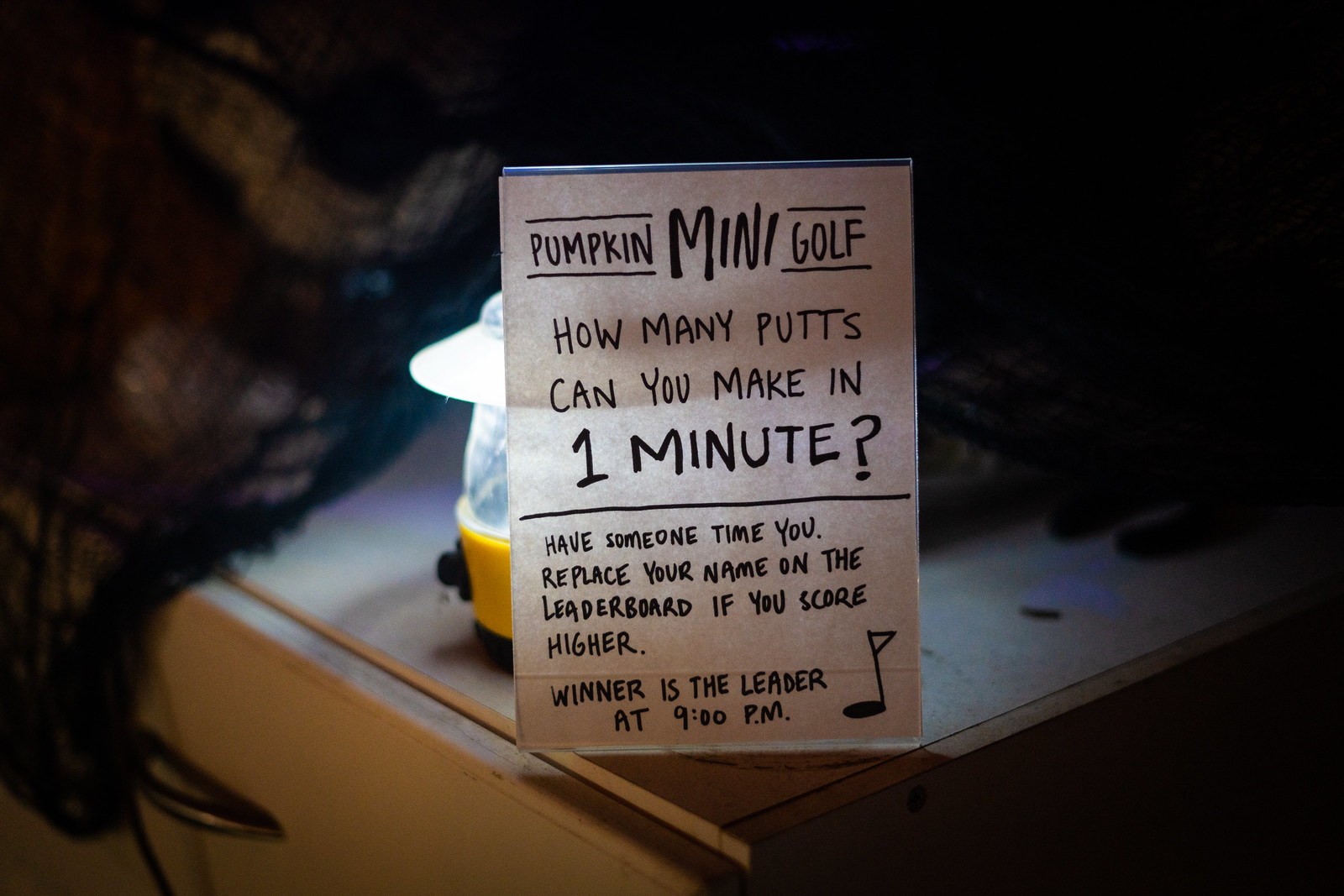This image features a brightly lit lantern positioned behind a small acrylic stand that holds a white note card with black text. The note enthusiastically announces "Pumpkin Mini Golf" and challenges readers with the question: "How many putts can you make in one minute?" Beneath this, it instructs participants to "have someone time you" and to replace their name on the leaderboard if they score higher. The ultimate challenge is to be the leader by 9 p.m. The card also depicts a drawing of a golf hole with a flag. The setup is situated on top of a white dresser with a silver-toned handle, which also holds a black article of clothing. To the upper left, a mesh laundry bag is visible. The overall scene is in a dimly lit room, adding a cozy yet competitive ambiance to the mini golf challenge.